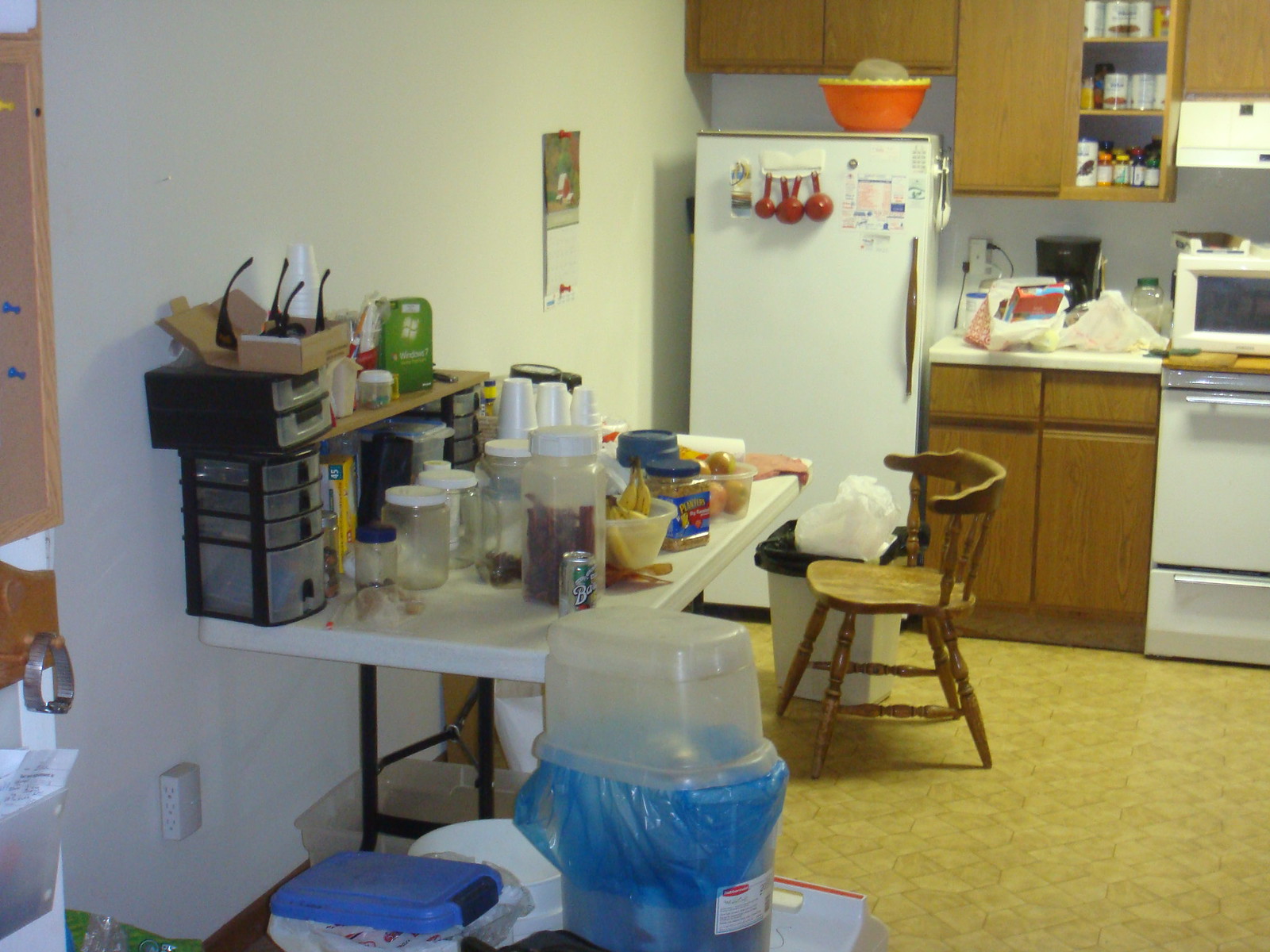The image depicts a somewhat cluttered and dated kitchen. On the left side, there is a fold-out table with various items, such as plastic drawers, a box of sunglasses, styrofoam cups, food containers, a canned drink, and several empty containers with white lids. On the floor below the table, there are additional plastic containers with lids, and a taller Rubbermaid container, which seems designed for wrapping paper but is repurposed to hold a blue recycled bag with a lid. 

In the background, there is a brown chair and a rectangular garbage can with both a black and white bag protruding from it. A white refrigerator is visible, featuring red measuring cups attached to its door. To the left of the refrigerator is a wall calendar. Atop the fridge sits a large orange and yellow bowl. The brown cabinets, which appear to be filled with various items, harken to an older kitchen design. 

The countertop is laden with items including a coffee maker, a plug with multiple extensions, and various bags. To the right, the white stove and exhaust fan are visible, completing the scene of this well-used, albeit disorganized, kitchen space.